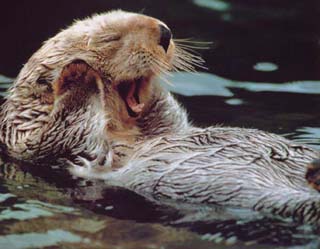In this captivating image, a very sleepy otter lies on its back, floating effortlessly in clear, greenish water. Its eyes are serenely closed, and its mouth is wide open in a visible yawn, revealing a pink tongue and two small teeth. The otter's furry paws are endearingly held up against its cheeks, emphasizing its relaxed demeanor. The otter’s fur is a blend of light brown, almost blondish hues on its head, transitioning to darker, wet fur on its body. Notably, its black snout is framed by prominent whiskers, adding character to its peaceful expression. The water around it reflects subtle ripples, complementing the otter's tranquil rest. This endearing scene captures the essence of the otter's serene moment, highlighting its tired yet contented state.